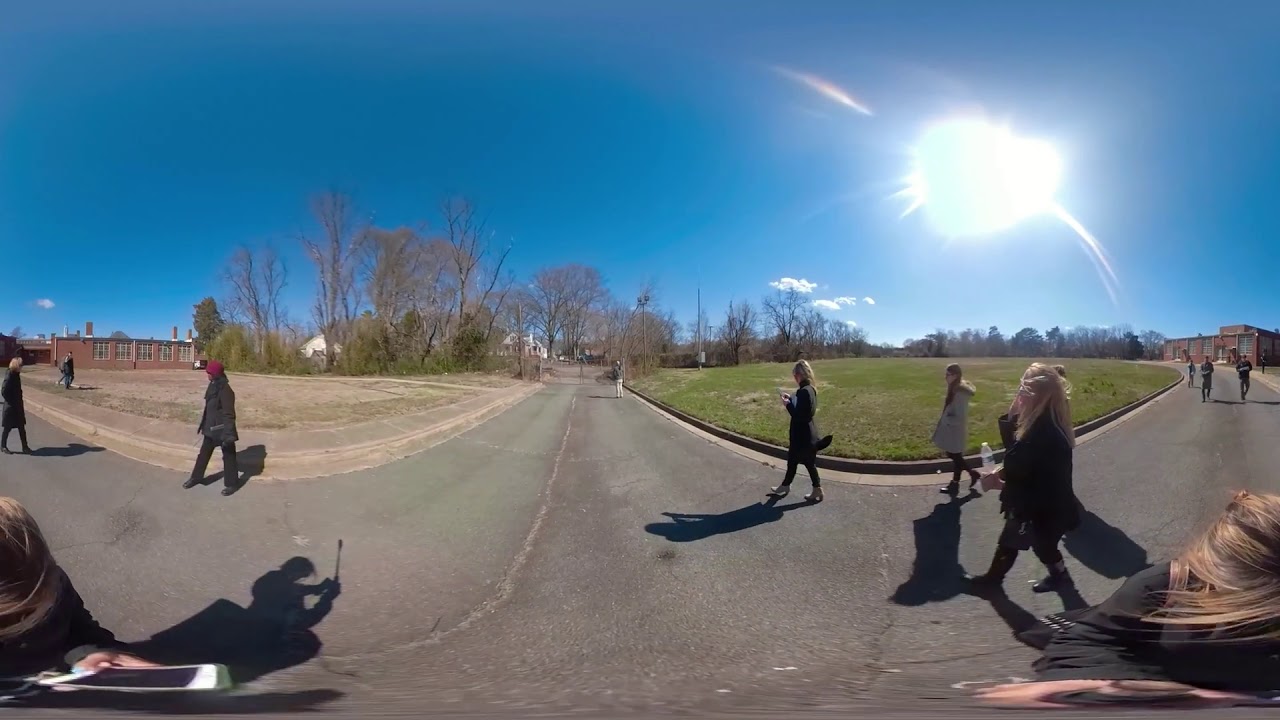In this panoramic image of a suburban park or campus, several groups of people are walking along a series of intersecting asphalt paths that form a 'W' shape. The scene is sunlit with a bright blue sky and a white, brilliant sun shining from the top right corner. The left side of the image showcases a brown brick building surrounded by parched, brown grass, and trees to its right. On the right, lush green grass and brown trees frame another brown building situated towards the middle of the right side. The paths are populated with people, possibly all white women, many dressed in winter clothes, moving in different directions. In the immediate foreground, the asphalt road extends from left to right, with another path stretching forward. In total, there are at least 12 people visible, providing a lively atmosphere despite the autumnal, somewhat neglected grassy areas. The far distance reveals additional trees and residential buildings partially hidden by the foliage.